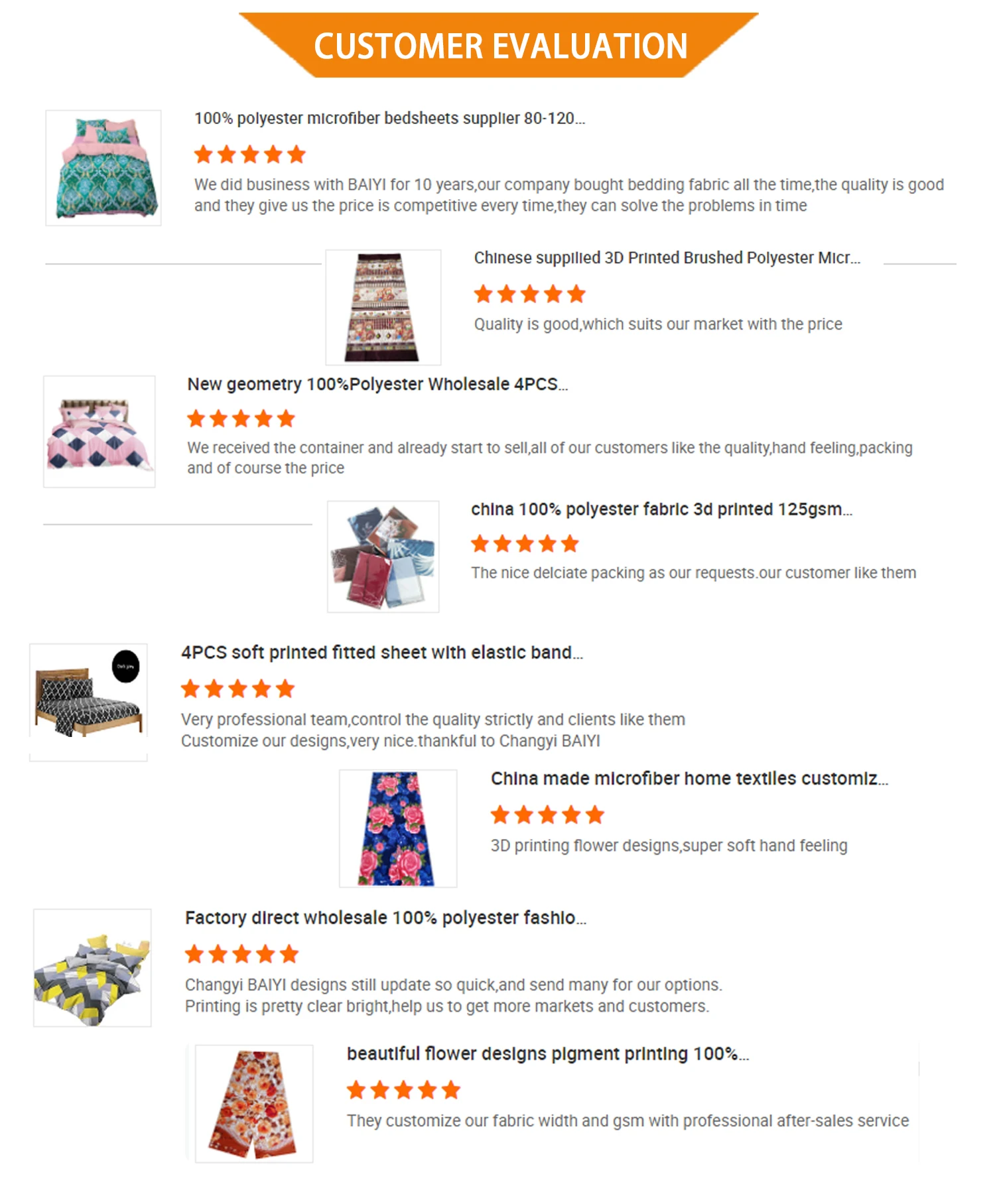The image appears to be a webpage, specifically dedicated to customer evaluations. At the top, there is an orange label with white text that reads "Customer Evaluation." Below this label, the page features various pictures, predominantly of bedding items. Each bedding image is paired with a detailed review. Each review consists of a title and a corresponding star rating. Notably, all the designs showcased have achieved a five-star rating. Beneath the stars, each review contains unique written feedback from different customers, reflecting their individual experiences and satisfaction with the bedding products.